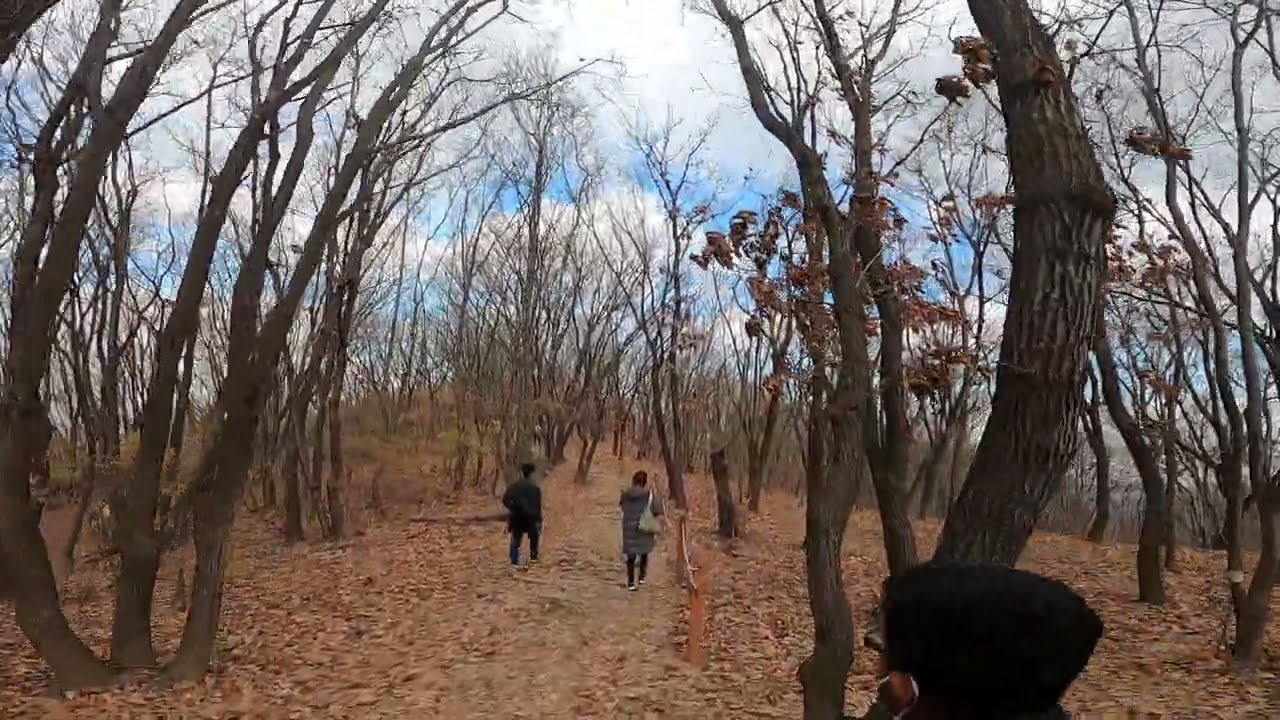The photograph captures a scenic autumn trail winding through a dense wooded area, where the trees have largely shed their leaves, blanketing the ground in a tapestry of brown and orange foliage. The late fall atmosphere is adorned with a bright blue sky peeking through sparse clouds, casting a crisp, cool light over the scene. Three hikers make their way along the path: A woman in the foreground, wearing glasses, a knit hat, and a face mask, with over-the-ear headphones doubling as earmuffs. To her right, a woman dressed in a dark gray puffy coat and black pants carries a beige purse slung over her shoulder. Beside her, a man in a black jacket and black pants completes the trio, with a black backpack visible on his shoulders. The distant curvature of the trees and branches hints at a fisheye lens effect, amplifying the immersive essence of this peaceful, chilly autumn hike.